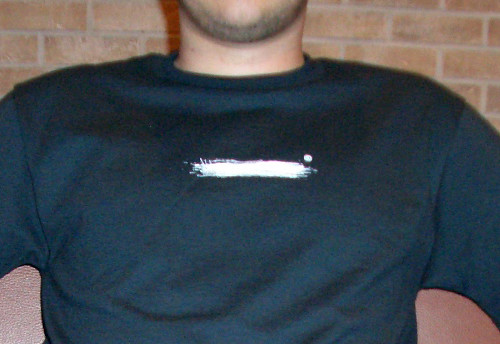In this detailed photograph, we observe a man whose face is mostly obscured, showing only the bottom of his chin with some dark stubble. His skin is light tan or pale. He is dressed in a dark-colored shirt—likely black—that displays a distinctive white paint-like design. This design features a small white dot over the top right of a painted line or strip located at the center of his chest. The shirt itself appears somewhat asymmetrical with one sleeve being baggier than the other. 

The man’s body is also presented in a somewhat asymmetrical manner. His head, including the top, is cut off in the photo, and only his chin, neck, chest, shoulders, and parts of his stomach and arms are visible. He stands or sits against a backdrop of a faded red-brown brick wall that has visible gray cement in between the bricks, giving a worn and aged appearance. Additionally, the background includes a maroon seat, and there appears to be a light source shining from behind the camera, casting light onto the subject.